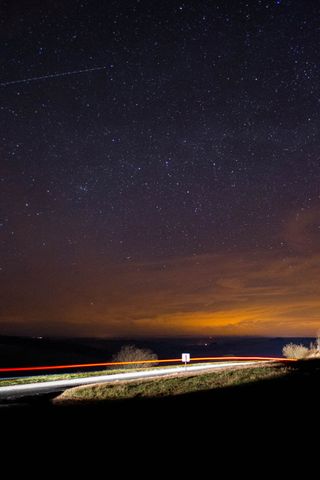The photograph captures a vivid night scene, showcasing an enchanting twilight transition in the sky. The upper portion is enveloped in near-black darkness, descending to a bluish-purple hue midway, and culminating in a golden-yellow glow close to the horizon—suggesting the sun has recently set. The land beneath is cloaked in shadow, punctuated by many white, star-like specks scattered across both the sky and terrain. Two prominent sources of white light, one to the left and another near the center, illuminate the darkened landscape.

In the foreground, a short stone wall is topped by an orange horizontal line, likely a metal fence, adding a structural element to the image. The road, possibly a highway, is faintly lit by what appears to be artificial light from an unseen source, perhaps car headlights, as implied by the orange streak possibly created through a time-lapse effect. A traffic sign stands on the roadside, positioned with its back to the camera, hinting at possible oncoming traffic from the right. Notably, a dotted line in the sky, resembling a shooting star or an artifact of time-lapse photography, runs through the star-dotted night, adding a touch of mystique to the tranquil, yet dynamic, scene.